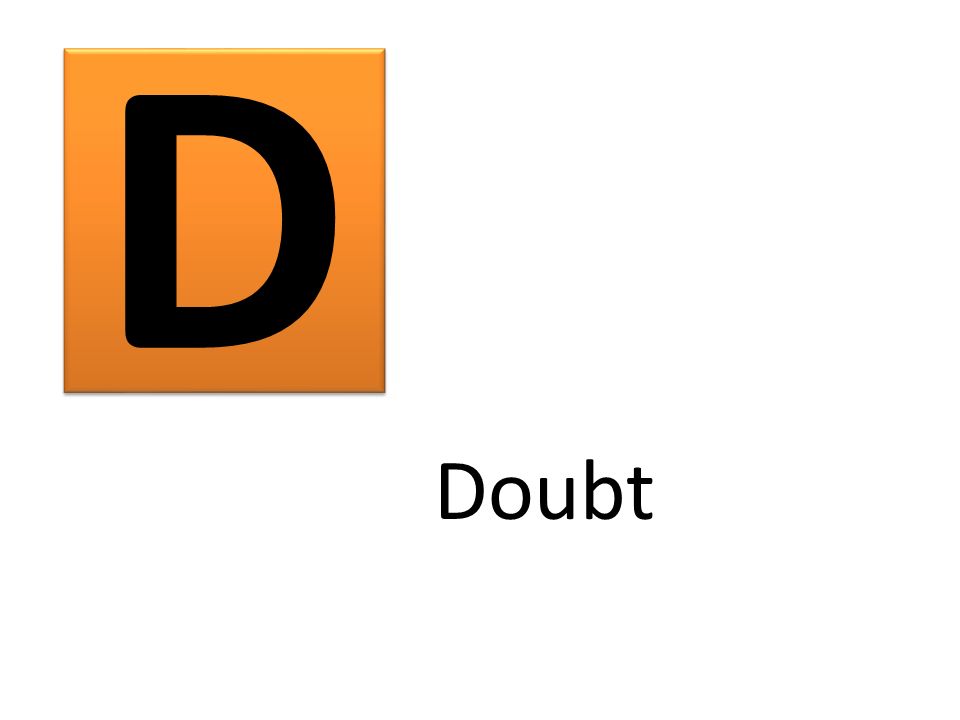The image features a plain white background with a slightly embossed, gradient orange rectangle (or square) in the upper left corner. The gradient varies from a brighter orange at the top to a slightly darker shade at the bottom. In the center of this orange shape, there's a prominent black capital letter "D", creating a subtle 3D effect as if raised off the background. In the lower right corner of the image, much smaller in size and rendered in a simple Courier New font, is the word "Doubt", with only the 'D' capitalized. The arrangement and elements give the impression of a flashcard, illustrating the letter "D" and its corresponding word "doubt".